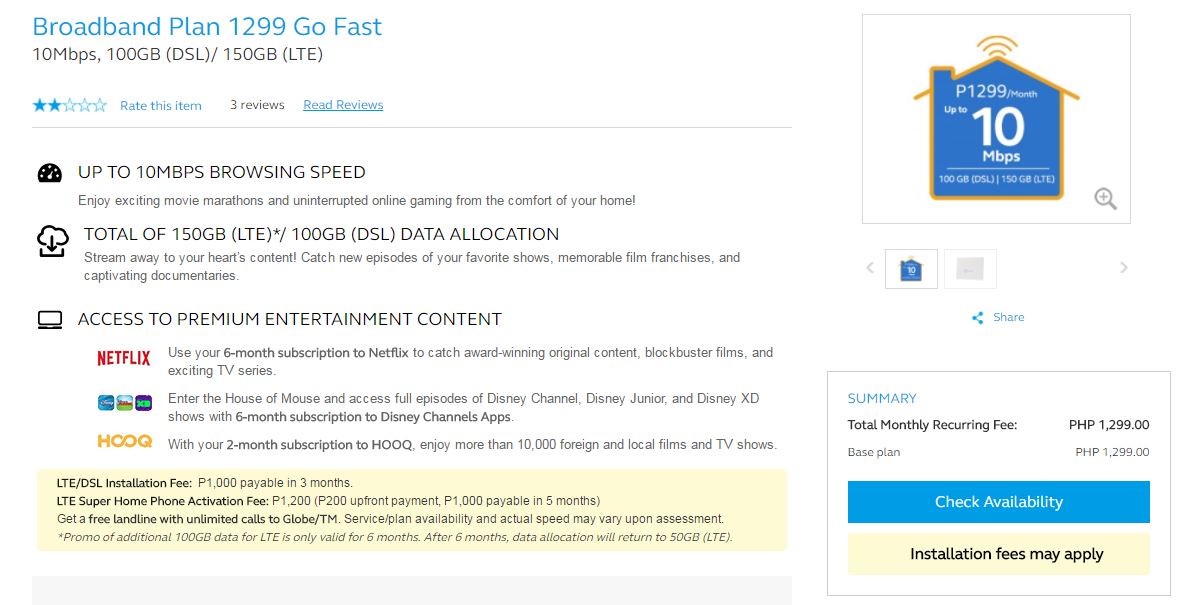The image is a detailed screenshot of a broadband plan advertisement, primarily rendered in a blue and pale yellow color scheme. At the top, in light blue text, it displays "Broadband Plan 1299 Go Fast." Below this, black text indicates the plan details: "10 Mbps, 100 GB (DSL) / 150 GB (LTE)."

The advertisement features a rating system where out of 5 stars, 2 are filled in. It invites viewers to "Read this item" with the note "3 reviews" underlined next to it.

Further down, it outlines the plan benefits: "Up to 10 Mbps browsing speed," "Total of 150 GB (LTE) / 100 GB (DSL) data allocation," and "Access to premium entertainment content" including Netflix. Three icon-filled squares beneath this show an "H," an infinity symbol, and a "Q."

In a pale yellow banner, the advertisement mentions additional fees: "LTE/DSL installation fee" and "LTE Super Home Phone activation fee." Adjacent to this is a square featuring a house icon with a blue background and yellow-orange trim, labeled "P1299 per month, up to 10 Mbps."

The bottom part of the advertisement provides a summary of costs: "Total monthly recurring fee: PHP 1299," "Base plan: PHP 1299," and a note stating "Check availability" with a reminder that "installation fees may apply."